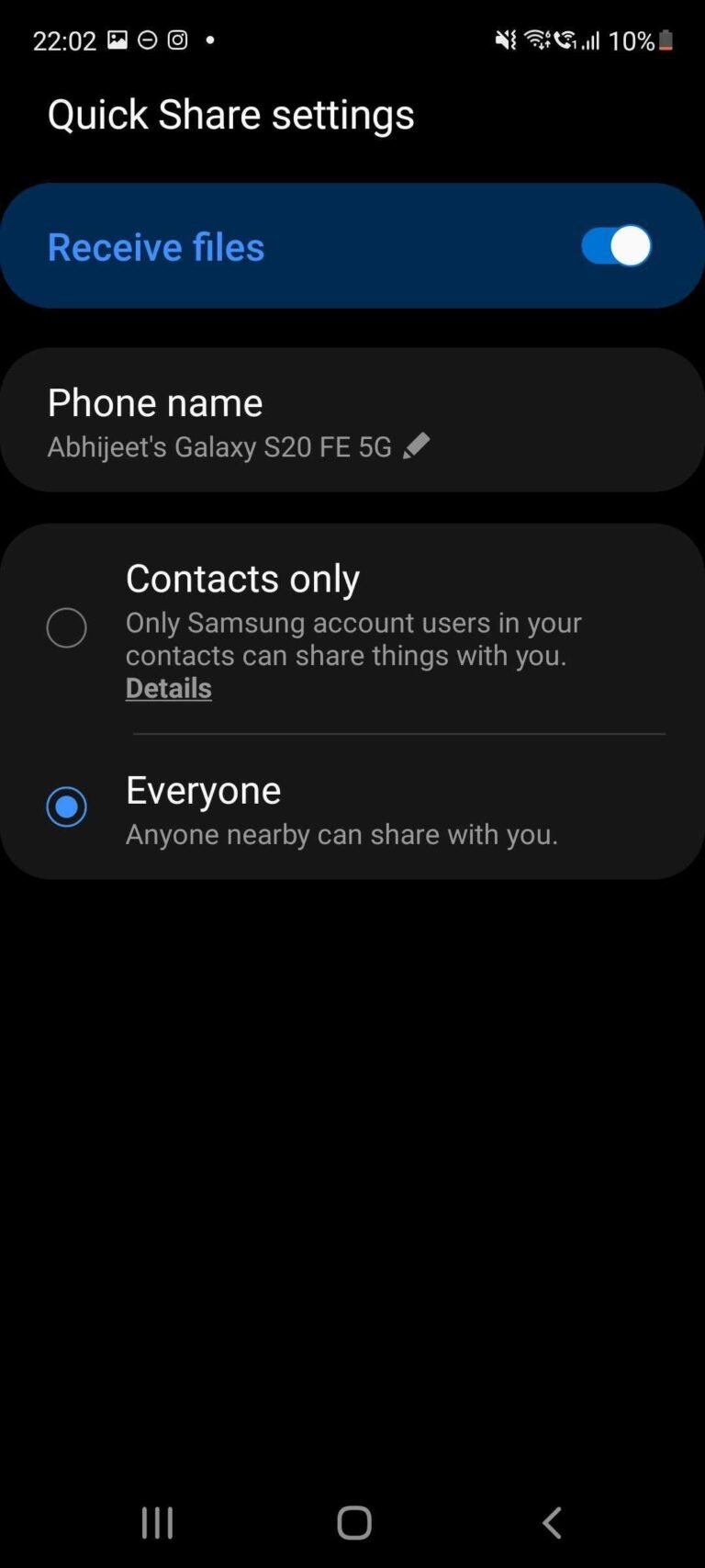**Detailed Caption:**

The image is a screenshot taken from a Samsung Galaxy S20 FE 5G smartphone at 10:02 PM with a low battery level of 10% and a weak signal indicator. The display shows the "Quick Share Settings" menu against a black background. The "My Files" option, highlighted on a blue background, indicates that it is active. Under the device name "Jit's Galaxy S20 FE 5G," the screen informs that sharing is currently set to "Contacts Only," allowing only Samsung account users in the contacts to share files.

Below this setting, the screen displays options for sharing details: the word "Details" appears with an unselected circular checkbox next to it, and a more prominent option, "Everyone," is visible with a blue-filled circular checkbox, indicating it is enabled. This setting permits anyone nearby to share files with the user.

At the bottom of the screen, the standard Android navigation buttons are visible: the "Close" button, the "Home" button, and the "Go Back" button, set against the customary layout. The background remains predominantly black, ensuring a clear and focused display of the options and settings described above.